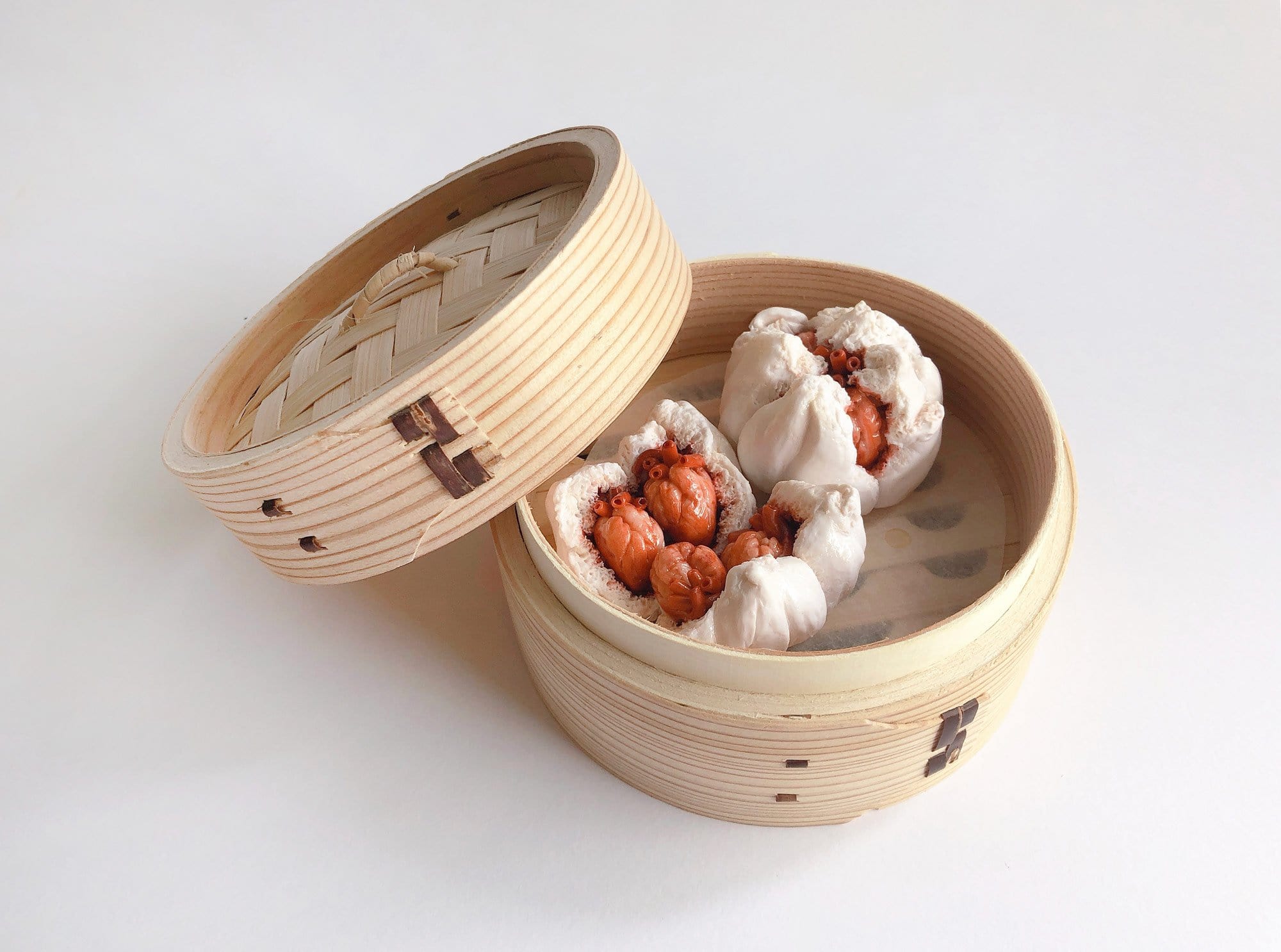This is a detailed and descriptive caption combining and emphasizing shared details from the observations:

In this intriguing image, we see a light bamboo or woven wooden basket, characteristic of those used for dim sum, open with the lid resting to the left. The basket is placed on a white surface with a subtle gradient, hinting at a light source coming from the right. Inside the basket, there are two pale, bread-like dumplings, which might be computer-generated. Both dumplings are split open, revealing several miniature hearts that appear unnaturally red and pristine, possibly resembling cleaned animal hearts. Despite their uncannily realistic appearance, these hearts seem to be crafted from a material akin to Play-Doh. The entire setup carries a surreal, almost unsettling quality, indicative of an AI-generated image where the hearts and dumplings themselves appear meticulously arranged, with some wooden meat or decorative item visible beneath the back dumpling, adding an additional layer of visual interest.